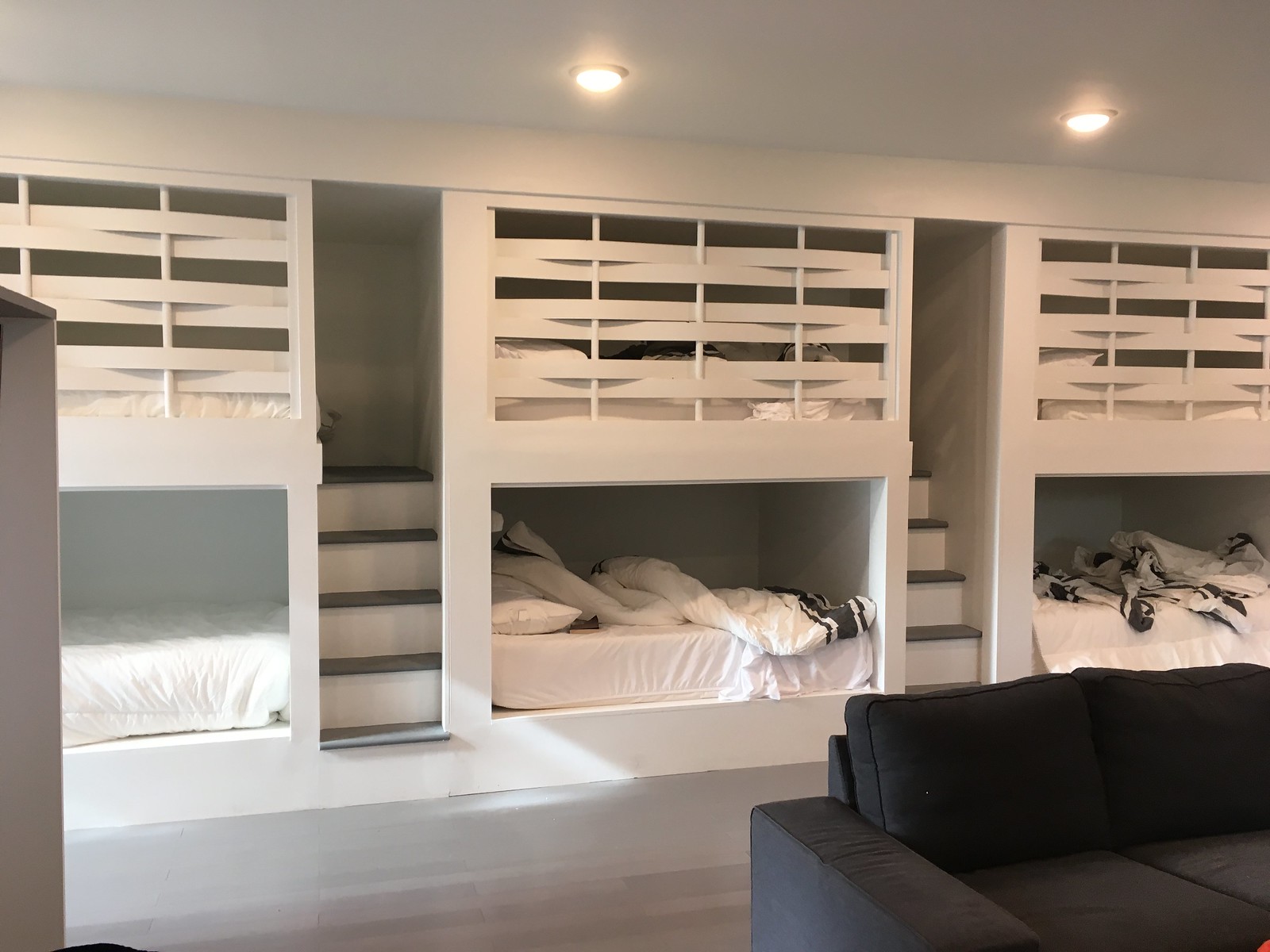The image depicts a brightly lit room with built-in, white bunk beds resembling sleep pods arranged neatly along the wall. There are three sets of bunks, each comprising a lower bunk that is open and an upper bunk that is semi-enclosed by a white latticework, likely intended to prevent falls and provide some privacy. Each bunk has standard bedding, including pillows, sheets, and blankets with white and black details. The upper bunks are accessed by small sets of white stairs with dark grey treads situated between the bunks.

In the foreground, a black couch with plush cushions faces the sleeping area. The floor appears to be light-colored linoleum, and the room is illuminated by inset ceiling lights and natural sunlight streaming in from the left side, suggesting a possible window not visible in the image. Overall, the setting evokes a dormitory-like atmosphere, potentially suitable for multiple occupants, such as in a hostel or a shared children's bedroom.